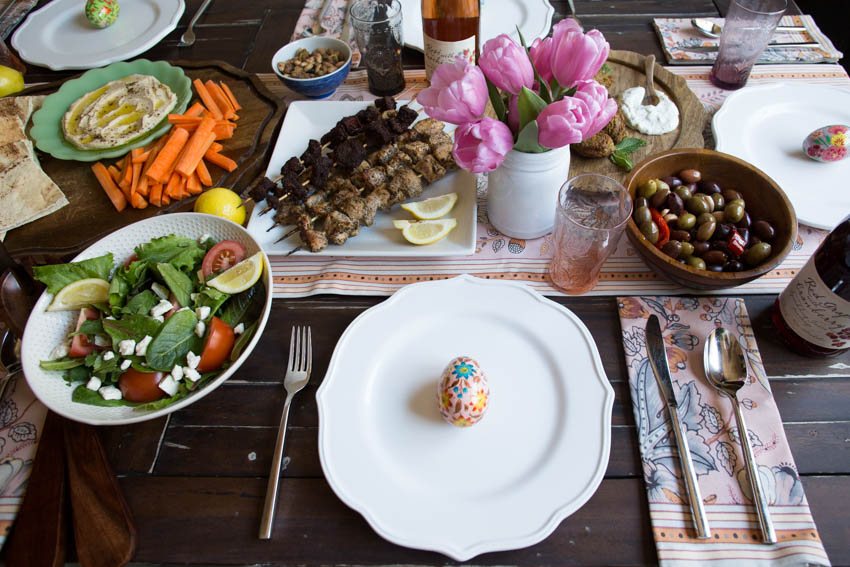The image presents a top-down view of a diverse and elaborate dining setup, likely at a sophisticated restaurant. At the center of a black table, there is a circular plate with intricate grooves around its edge, holding a single, decorative Easter egg. To the right of this central plate lies a pink napkin adorned with brown stripes on its bottom third and a floral design, flanked by a knife on the left and a spoon on the right. Next to this setup, without any napkin, is a fork placed to the left. Adjacent to the fork, there is a vibrant salad bowl featuring fresh lettuce or spinach leaves, tomatoes, lemon slices, and a sprinkling of cheese. Above the spoon, a smaller bowl contains a mix of pickles and black raisins.

On the right side, there's a wine bottle beside another diner's setting, complete with an empty glass. Dominating the table's center is a decorative bowl filled with pink flowers. To its right, a dish of cooked sausages with a side sauce is visible. On its left, a square plate holds skewered meats, likely beef and lamb, accompanied by lemon slices. In the top left corner, there is another small bowl cradling an egg, and below it, an egg dish with carrot slices. Scattered throughout the table, various white plates and fine silver cutlery add to the elegant dining experience. The assortment of dishes, vibrant hues, and carefully arranged details create a visually rich and colorful scene against the sophisticated backdrop of a dark table.